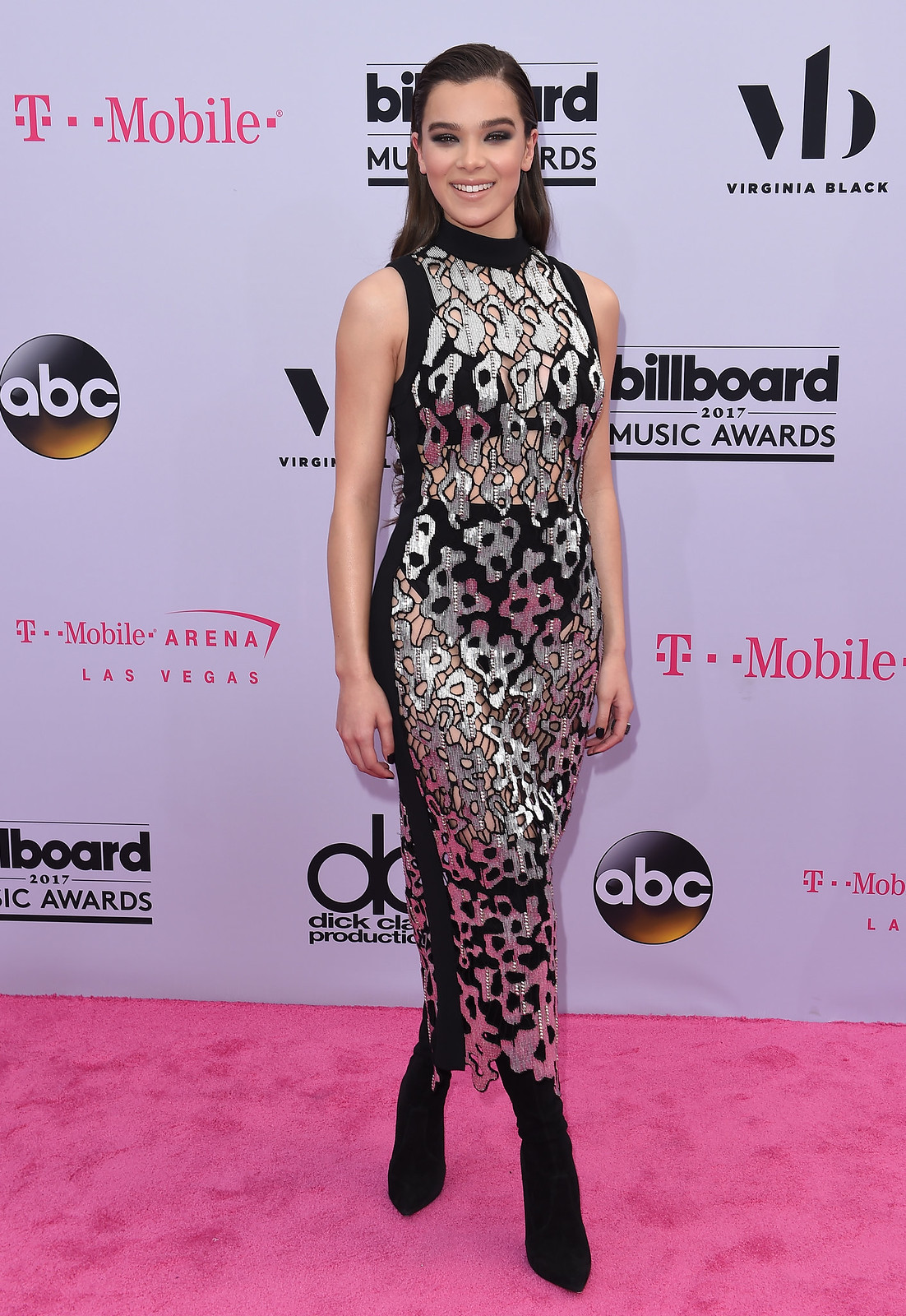In the photograph, a young Caucasian woman with dark brown, slicked-back hair stands on a pink carpet, which occupies about a quarter of the image at the bottom. The photograph is taken in portrait mode, making it taller than it is wide. The pink carpet is slightly fuzzy, higher on the left, and slopes downward to the right.

She is posing confidently with her legs crossed and her arms hanging at her sides, smiling directly at the camera. She appears to be in her late teens or early 20s. The woman is wearing a sleeveless silver metallic dress with black borders, which is distinctly see-through and patterned in a way that resembles leopard print, revealing her black underwear underneath. Her footwear consists of black boots.

The background is adorned with a light-colored wall featuring numerous brand logos and names. Prominently displayed are "T-Mobile" in pink text at the top left, "Virginia Black" with its VB logo in black text at the top right, "ABC" in white text within a black circle on the middle left, and "Billboard Music Awards" along with "T-Mobile Arena Las Vegas" in various spots. The visible signage underscores the event context, suggesting that this is a high-profile show or music awards ceremony.